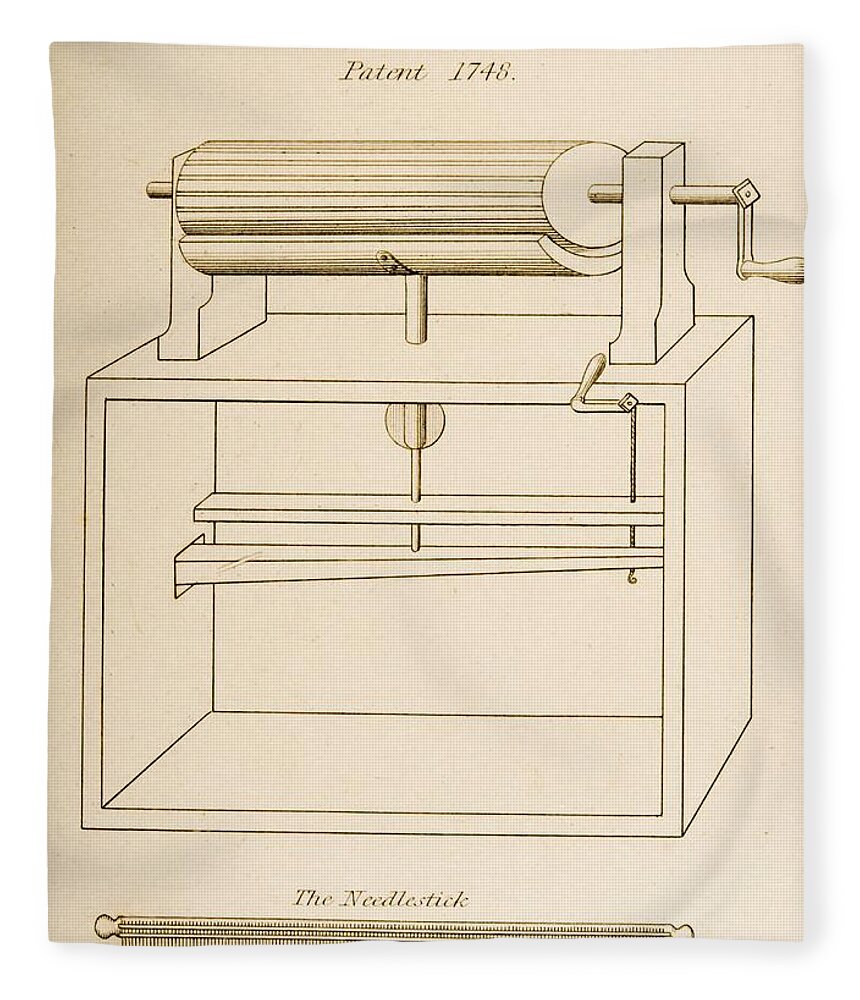This image showcases a detailed drawing from Patent number 1748, clearly labeled at the top. The drawing appears to be set against a quilted-looking background and depicts a mechanical device involving a cylindrical, hand-crank-operated mechanism. This cylinder is connected by an axle and crank, allowing for rotation. Below the cylinder, the illustration features a box housing additional mechanisms, including a small hanging chain that threads through a plank. Attached to this setup is a needle-like piece of metal that moves vertically when the rotary arm is engaged. At the bottom of the image, partially cut off, are the words "the needle stick," suggesting the device is related to sewing or textile operations. The mechanism seems designed to facilitate some mechanical process in fabric or cloth production.